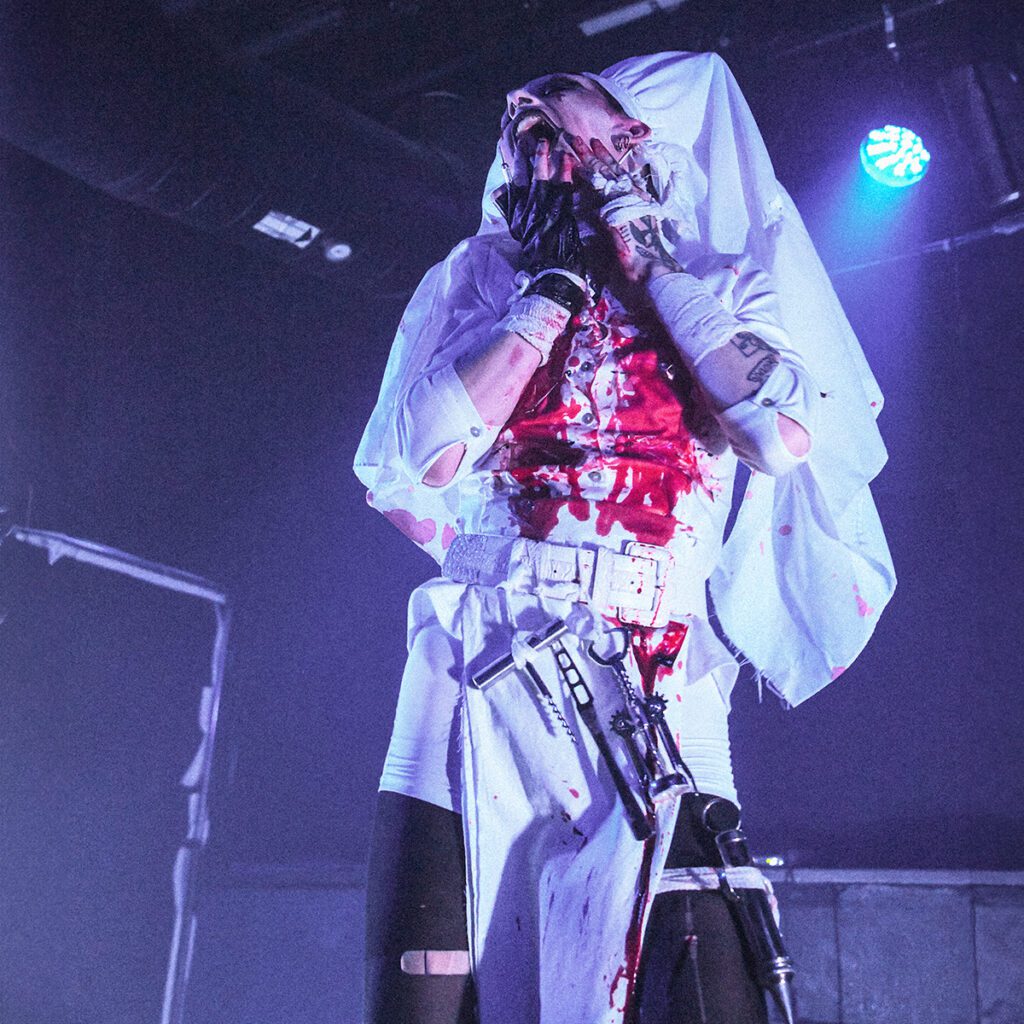This photograph captures a performer in mid-performance on an elevated stage, viewed from an audience's perspective, with the angle making the scene even more dramatic. The individual, likely a woman, exudes an eerie and medieval aura, blending elements of both horror and historical attire. She is dressed in a strikingly white nurse-like costume, which is gruesomely splattered with fake blood, creating a stark and shocking contrast. Her head is adorned with a medieval-style pointed hat, complete with a flowy scarf fabric draping around it, reinforcing the period look. Her makeup enhances the gothic atmosphere, featuring a pale face with black-outlined eyes and lips. Additionally, she wears black fingerless gloves on her right hand, while her left forearm is covered in tattoos. The white tunic top is fastened with a white belt, from which various instruments—perhaps surgical or torturous—dangle ominously. Black leggings peek out from beneath her tunic, completing her disconcerting ensemble. The setting appears to be a blackout theater with a spotlight illuminating her, heightening the dramatic effect of what seems to be a gory play or a haunted house attraction. Her intense expression and upward gaze suggest she might be in the midst of delivering a chilling scream, adding to the overall macabre mood of the scene.